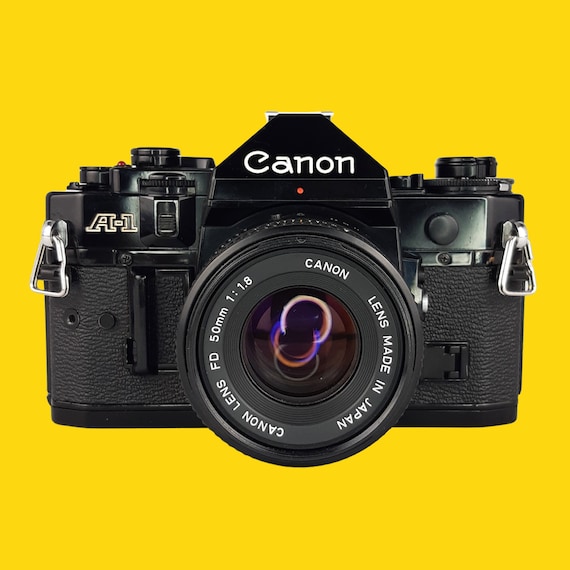The image depicts a vintage black Canon film camera set against a stark yellow background. Dominating the center is a detailed Canon lens with smooth glass reflecting colorful rings of pink, blue, and red, likely due to ring lights used in the photographic setup. The lens, inscribed with white text, reads "Canon lens FD 50mm 1:1.8" and "Lens made in Japan." The camera's body features the iconic "Canon" logo prominently in the middle, accompanied by a small red dot just below it. On the upper left-hand side, in raised white lettering, is "A1," adjacent to a metal connector for camera straps, mirrored on the right side as well. The camera boasts a textured grip area and various buttons, knobs, and dials atop its structure, indicative of its old-school, hands-on operational style. The overall composition, complete with silver clips on the edges, highlights the camera's meticulous design and robust functionality.